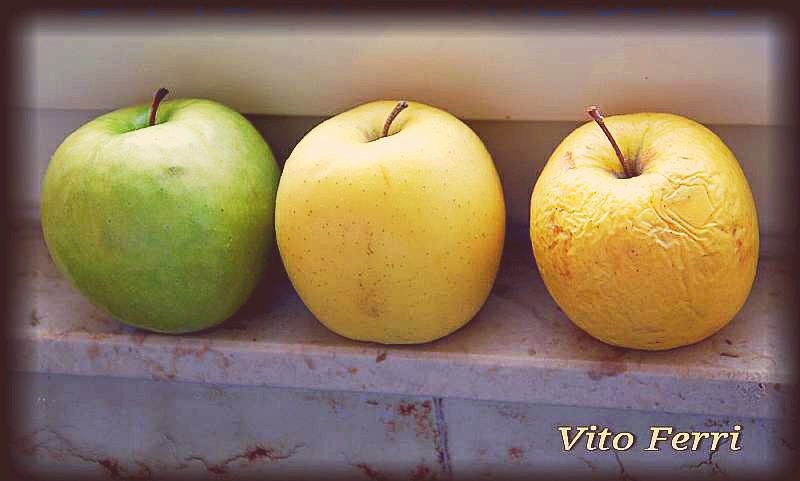This painting, oriented landscape, depicts three apples placed on a staircase with a marble appearance, where the marble features a striking red hue against a primarily gray-white background. The first apple on the left is a crisp, green Granny Smith apple, followed by a yellow apple with faint speckled brown dots in the middle. The third apple on the right is a weathered yellow apple with an orange tint, exhibiting signs of over-ripeness through its wrinkled skin and markings. Each apple retains its small stem. Situated on a ledge that varies between beige and grayish tones with red streaks, the detailed artwork is signed in the bottom right corner with the creamy white text reading "Vito Ferri."